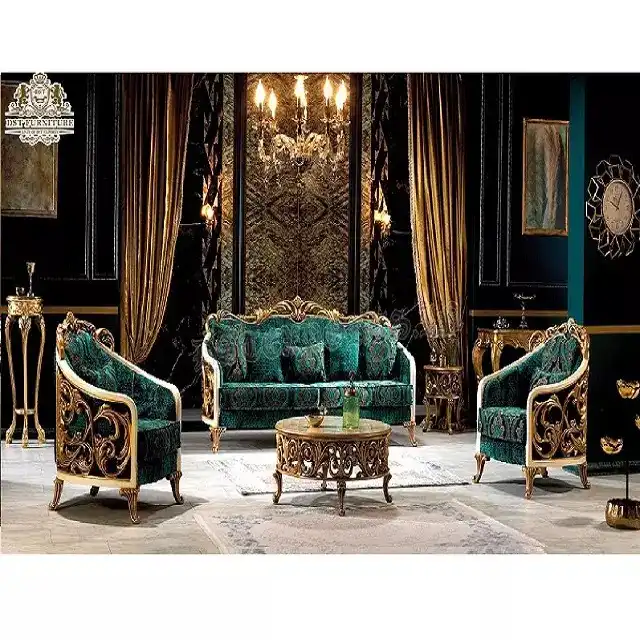The image showcases an opulent Victorian-era room that exudes high-class elegance, reminiscent of a royal palace or a luxurious showroom. The setting features a lavish sitting area dominated by rich gold and deep green hues. At the center, two ornate chairs with turquoise green upholstery face each other across a round, gold-finished coffee table. A matching Victorian-style loveseat, possibly accommodating two to three people, stands behind the table. The room is embellished with gold-framed paintings and large, bunched gold curtains that lend an air of grandeur. 

The walls are painted a deep jungle green, enhancing the room's regal atmosphere. Intricate tapestries adorn the walls alongside sconces designed to look like antique candle holders. The ceiling boasts a striking gold chandelier with six lights. To the right side, a silver and black clock adds a touch of modern contrast. Persian and grayish-white rugs enhance the plush feel of the space.

A smaller gold table on the left holds what seem to be silver cups, while decorative items such as a green bottle and a bowl sit on the coffee table. The image also contains an indistinct label in the upper left corner, possibly reading “DST Furniture,” hinting that this might be an advertisement for a high-end furniture collection.